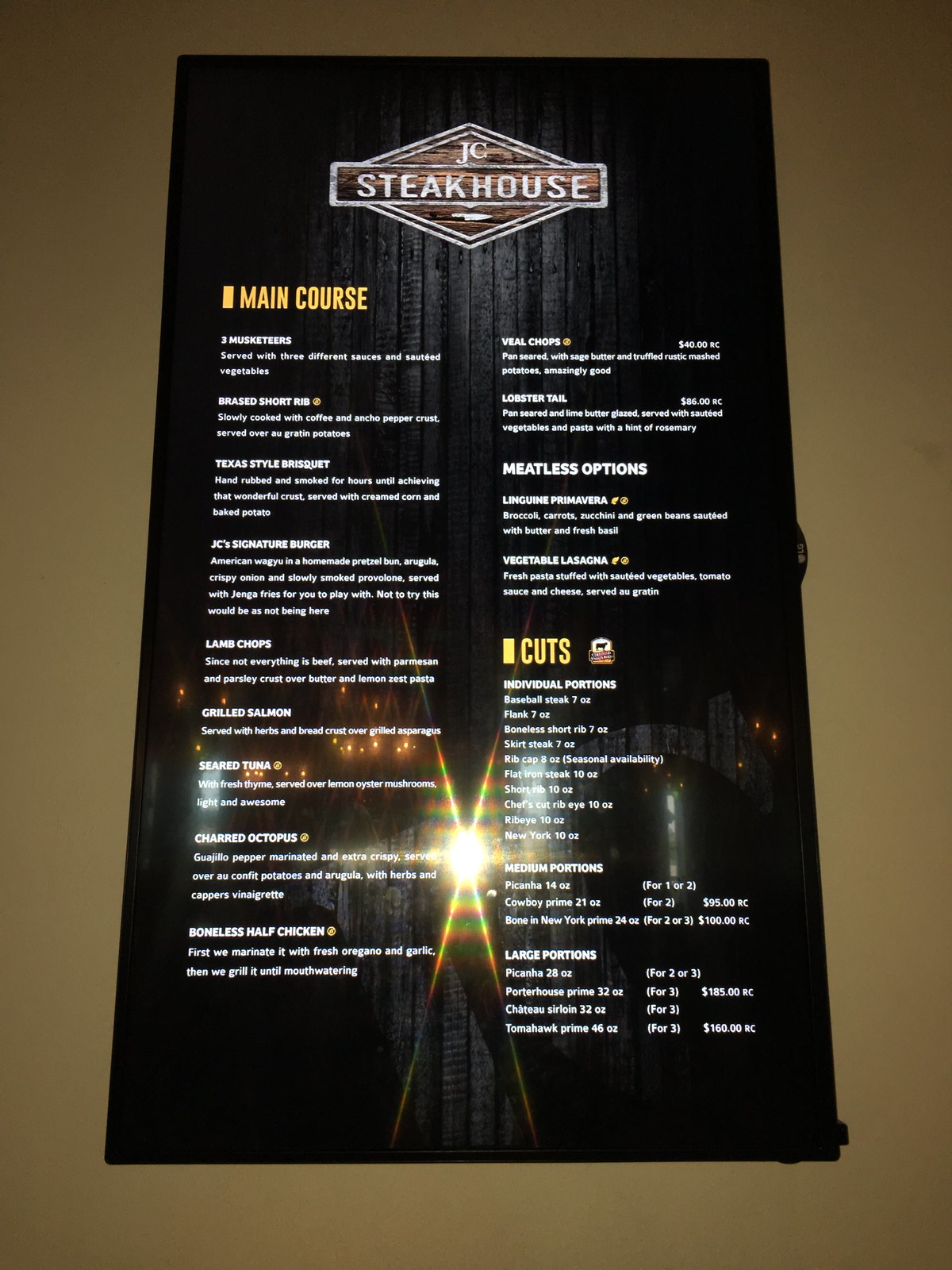A slightly blurry photograph depicts what appears to be a menu from JC Steakhouse. The menu, featuring a dark, sleek design that could either be a wood finish if it's mounted on a wall or a vinyl material if it lies flat on a table, is set against an entirely white background. This makes it challenging to discern whether the surface is indeed a wall or a table. 

At the top of the menu is the restaurant's insignia and the name "JC Steakhouse," written in distinctive lettering. Below this, the menu lists a variety of main courses, although the finer details are difficult to read due to the small font. Some of the legible headings include enticing dishes such as "Texas-Style Something," "Grilled Salmon," "Lamb Something," "Charred Octopus," and "Boneless Half Chicken." 

Each dish has brief descriptions in tiny print underneath, rendering them almost unreadable. There is also a visible section dedicated to "Veal Chops," and another section labeled "Meatless Options." Towards the bottom of the menu, there's a section titled "Cuts," presumably listing various types of steaks.

The image is slightly marred by the visible flash from the camera, which creates a reflective glare in the middle of the menu, accompanied by some light reflections in the background.